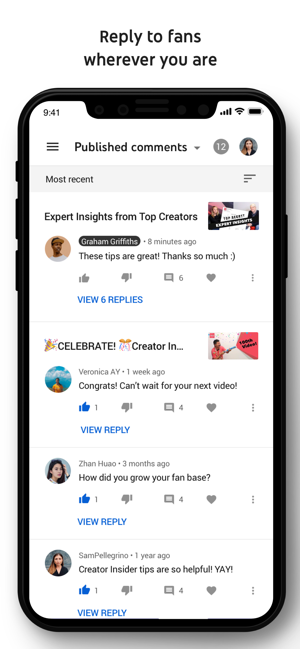A screenshot highlights an online interaction on a mobile interface. At the top, the phrase "Reply to fans wherever you are" is prominently displayed in black text. Below this, an image of a smartphone displays a website with a detailed layout. The time on the phone reads 9:41. A profile picture of a woman is located near a hamburger menu on the left side.

The screen shows sections for published comments, marked by an icon encircled with the number 12. There's a segmentation labeled "Most Recent," accompanied by a graphical representation of three ascending bars, each longer than the one below. The longest, top bar is captioned with "Expert insights from top creators," though the text is too small to be clearly read.

A recent comment by a male profile, posted eight minutes ago, reads, "These tips are great, thanks so much!" This comment has a reply icon indicating six available replies in blue text.

Another interaction, from a week prior by a user named Veronica A., includes a profile picture (likely of a man), stating, "Congrats, can't wait for your next video." This comment is marked with a thumbs-up icon bearing the number 1 and a comment icon showing 4 replies.